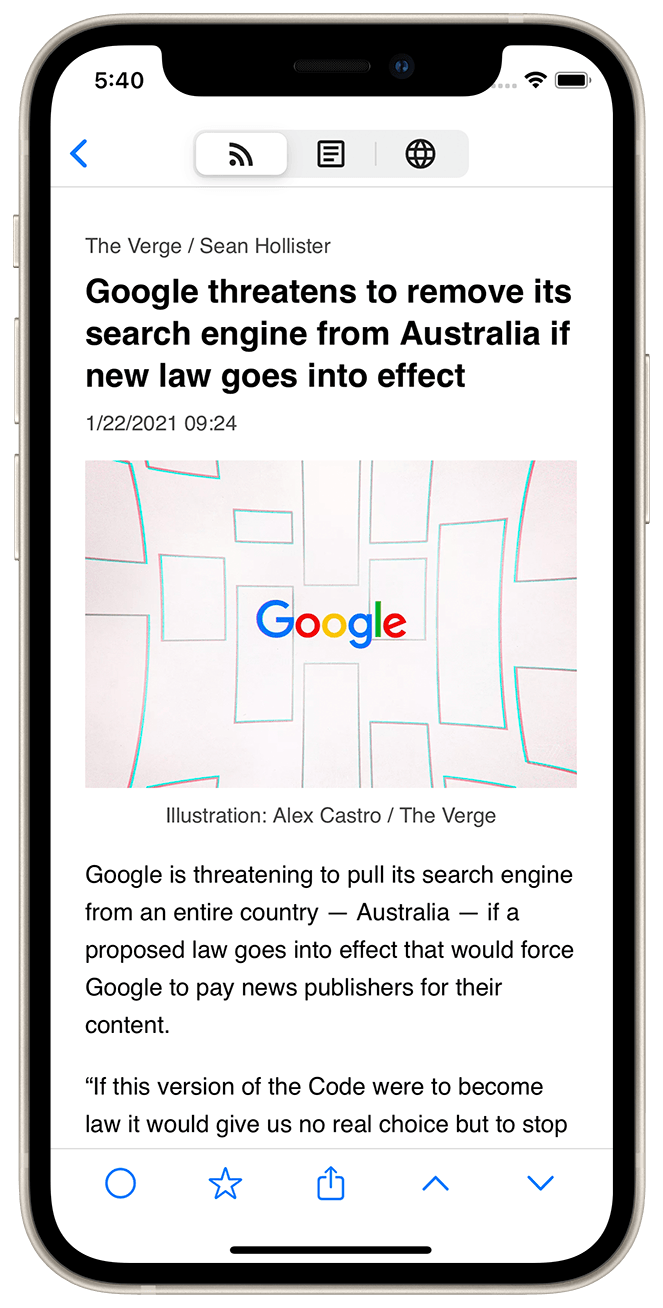The image depicts a smartphone encased in a white protective cover. The case features three buttons on the left side and a longer button on the right. At the top of the phone, the camera lens is visible. The time displayed on the screen is 5:40, and the device shows a full battery charge with an active Wi-Fi connection. 

The center of the screen shows a news headline from The Verge, written by Sean Hollister, which reads, "Google threatens to remove its search engine from Australia if new law goes into effect." The article was posted on January 22, 2021, at 9:24. Beneath the headline is an illustration credited to Alex Castro from The Verge, which features the Google emblem amidst various rectangles of different shapes and sizes. 

Accompanying text below the image explains, "Google is threatening to pull its search engine from an entire country, Australia, if a proposed law goes into effect that would force Google to pay news publishers for their content. If this version of the code were to become law, it would give us no real choice but to stop..." The message is cut off at this point.

At the bottom of the screen, several icons are aligned in a row, including a circle, a star, a download button, and an up arrow followed by a down arrow.